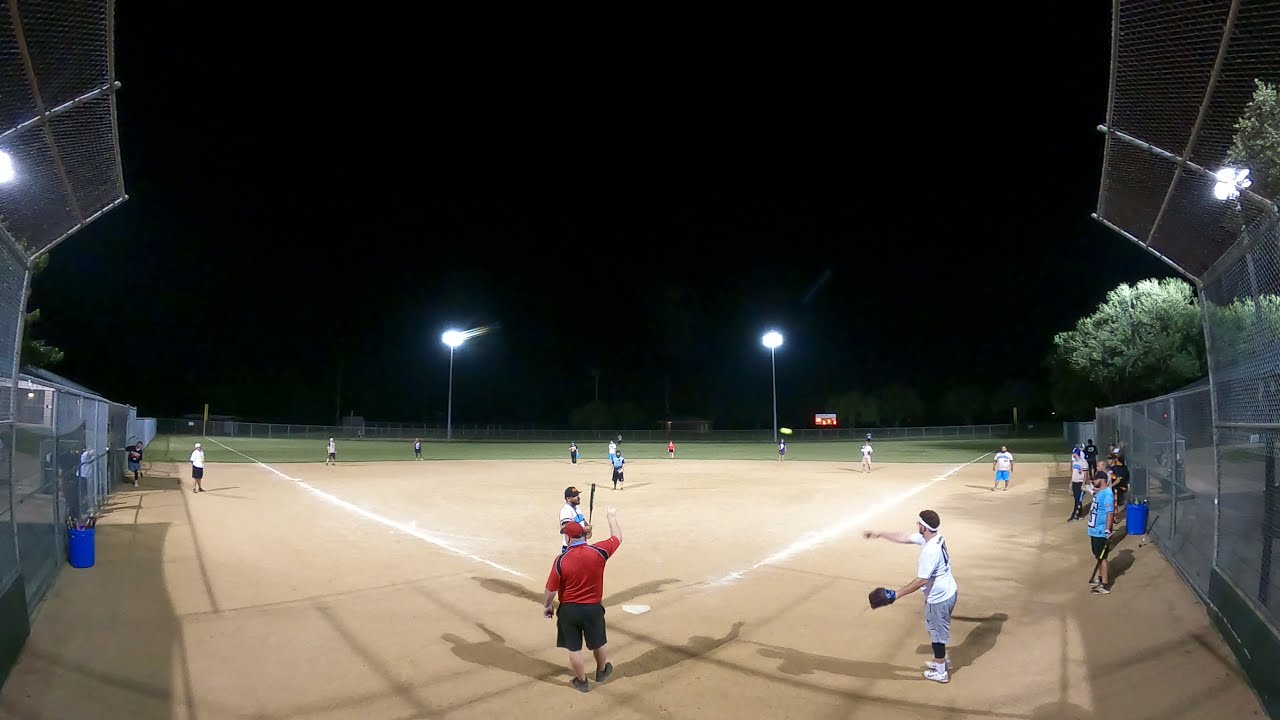The photograph captures the intense atmosphere of a nighttime baseball game from the perspective behind home plate. The pitch-black sky is starkly contrasted by the bright floodlights strategically placed behind the outfield, which cast strong illumination across the field. A batter from the white-uniformed team stands ready at home plate, gripping his bat and facing the pitcher. Positioned directly behind the batter is the umpire, identifiable by his red shirt, red baseball cap, and black shorts. To the right of the umpire stands the catcher, distinguishable by the mitt and white shirt.

The field itself is well-defined, with the sandy diamond clearly visible along with the home plate. Fencing cages flank both the first and third baselines, leading up to the dugouts. The fencing extends slightly over toward home plate on each side, encapsulating the play area. Down the first and third baselines, coaches can be seen guiding their teams, while clusters of players—both on the field and waiting near the dugout along the fence—immerse themselves in the game. Trees frame the right side of the field, their silhouettes visible beyond the fence, adding a touch of nature to the bustling scene. A background sign, likely from a high school, glows with an indistinct red hue. Additionally, a blue bucket and shadows cast by the fencing add to the intricate details of the setting. The overall scene encapsulates the structured chaos and excitement unique to a night game under the lights.